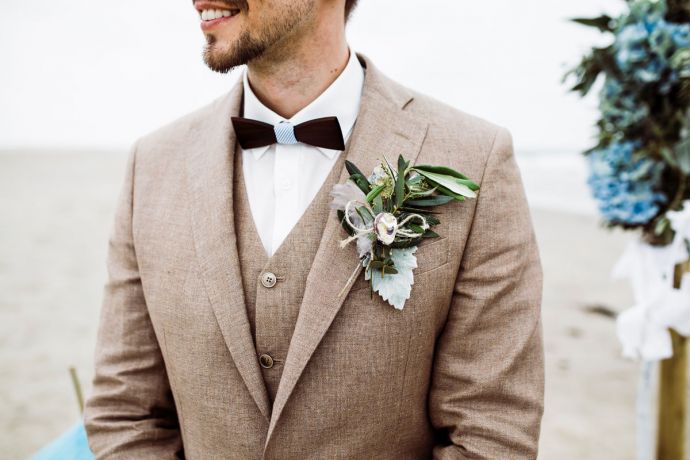In this color photograph taken at a beachside wedding, the partial view captures a groom from the chin down to his stomach, revealing his dark gray tweed three-piece suit adorned with a black bow tie. He wears a camel-colored vest under a brown jacket and a white button-up shirt. A corsage, featuring twine ribbon tied in a bow, green and olive leaves, a pink flower, and hints of blue and white, is pinned to his left pocket. The man's light beard, mustache, and goatee are closely cropped, and he is smiling, with his mouth slightly open, revealing his upper row of teeth. The background shows a sandy brown beach and blurry seawater. He stands near a makeshift altar framed with blue flowers, green leaves, and white ribbons, ready for the ceremony.